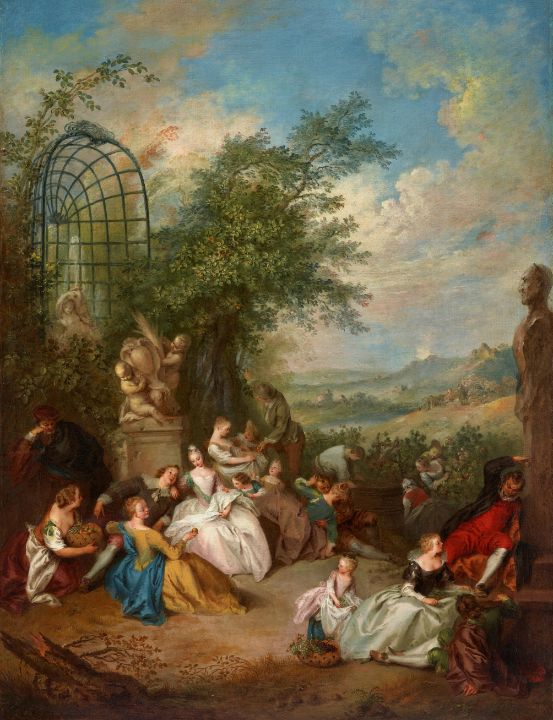This oil painting, likely from the Renaissance period and resembling something you'd find in a museum, depicts a lively and detailed scene during a grape harvest festival. Dominated by a vertical composition, the vivid and realistic artwork portrays men, women, and children dressed in elaborate, colorful gowns and suits, sitting and conversing on the dirt ground among several stone sculptures. Prominently on the right side stands a tall statue of a man facing left, while on the left side, two naked cherubic children grasp a vase, forming another sculpture. An additional statue of a woman is situated under an open, arched cage-like structure. The background features rolling fields and trees, all under a serene blue sky dotted with fluffy white clouds, which adds depth and tranquility to the festive gathering scene.